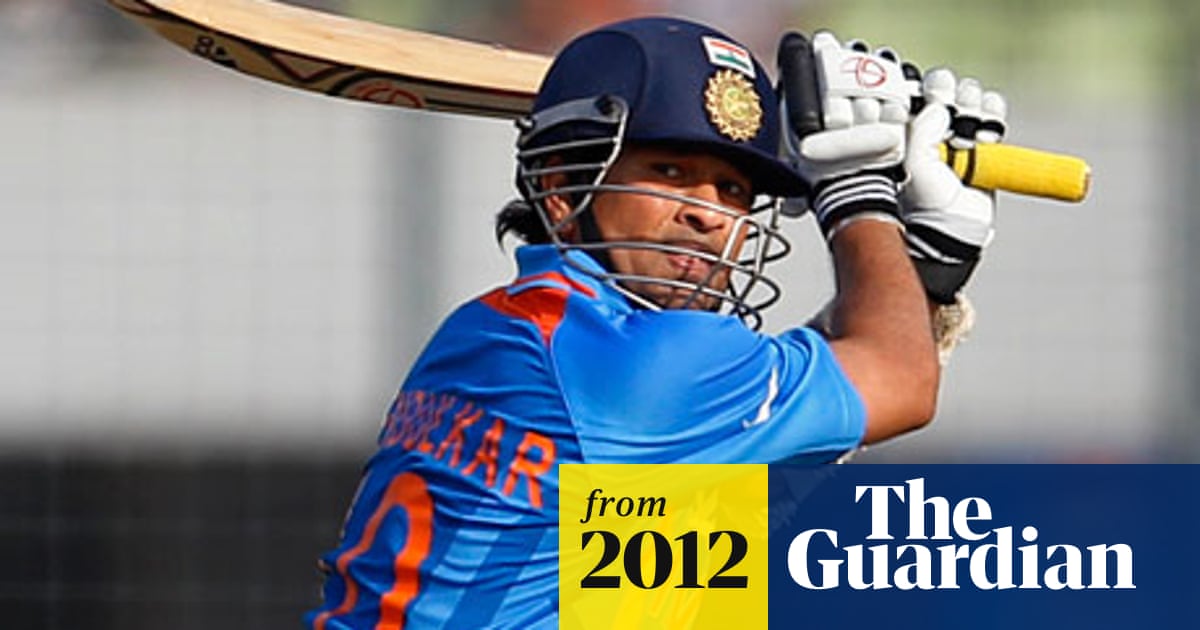The landscape photograph captures a man with dark skin, possibly of Indian descent, holding what appears to be a wooden cricket bat with a yellow handle near his gloved hands. He wears a navy blue helmet with a faceguard, matching white and black gloves, and a blue jersey that features orange text and numbers on the back, including a '0'. The jersey also sports vertical stripes and additional orange detail near the collar. The background of the image is a blurred mix of white, black, green, and orange hues. In the lower right-hand corner, there is a yellow box with black text stating "from 2012" and to its right, a dark blue rectangle with white text reading "The Guardian." The man is positioned facing to the right, but his head is turned towards the camera, creating a direct and engaging portrait.